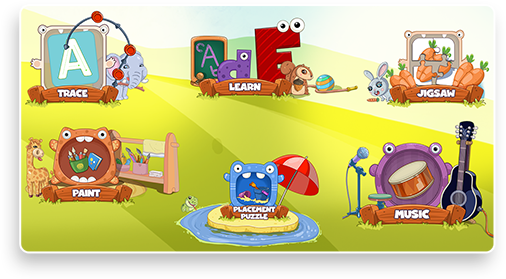This is a detailed description of a left-to-right horizontal image from a children's educational game typically found on a computer or smart device. The background features various shades of green designed to resemble grass, with lighter and darker strips creating a pattern that lightens as it recedes into the distance. In the foreground, there is a mound or hill, colored in yellow and green, set against a sky that has an ombre effect transitioning from blue to white, with darker blue in the middle fading to lighter shades at the edges.

In the main game interface, six distinct picture icons are displayed, each representing a different activity, accompanied by descriptive words in white text. 

- **Upper Left:** A large letter "A" with an elephant peeking around it, labeled "Trace."
- **Below Trace:** An art supply box featuring a giraffe, labeled "Paint."
- **Upper Middle:** The word "Learn" is displayed among letters with googly eyes and various animals.
- **Below Learn:** A garden scene with carrots and a rabbit, labeled "Jigsaw."
- **Middle Center:** A beach scene with an umbrella, labeled "Placement Puzzle."
- **Lower Right:** Musical instruments including drums, a guitar, and a microphone, labeled "Music."

The interface is clearly designed to provide a fun and interactive educational experience for young children, encouraging learning through various themed activities.